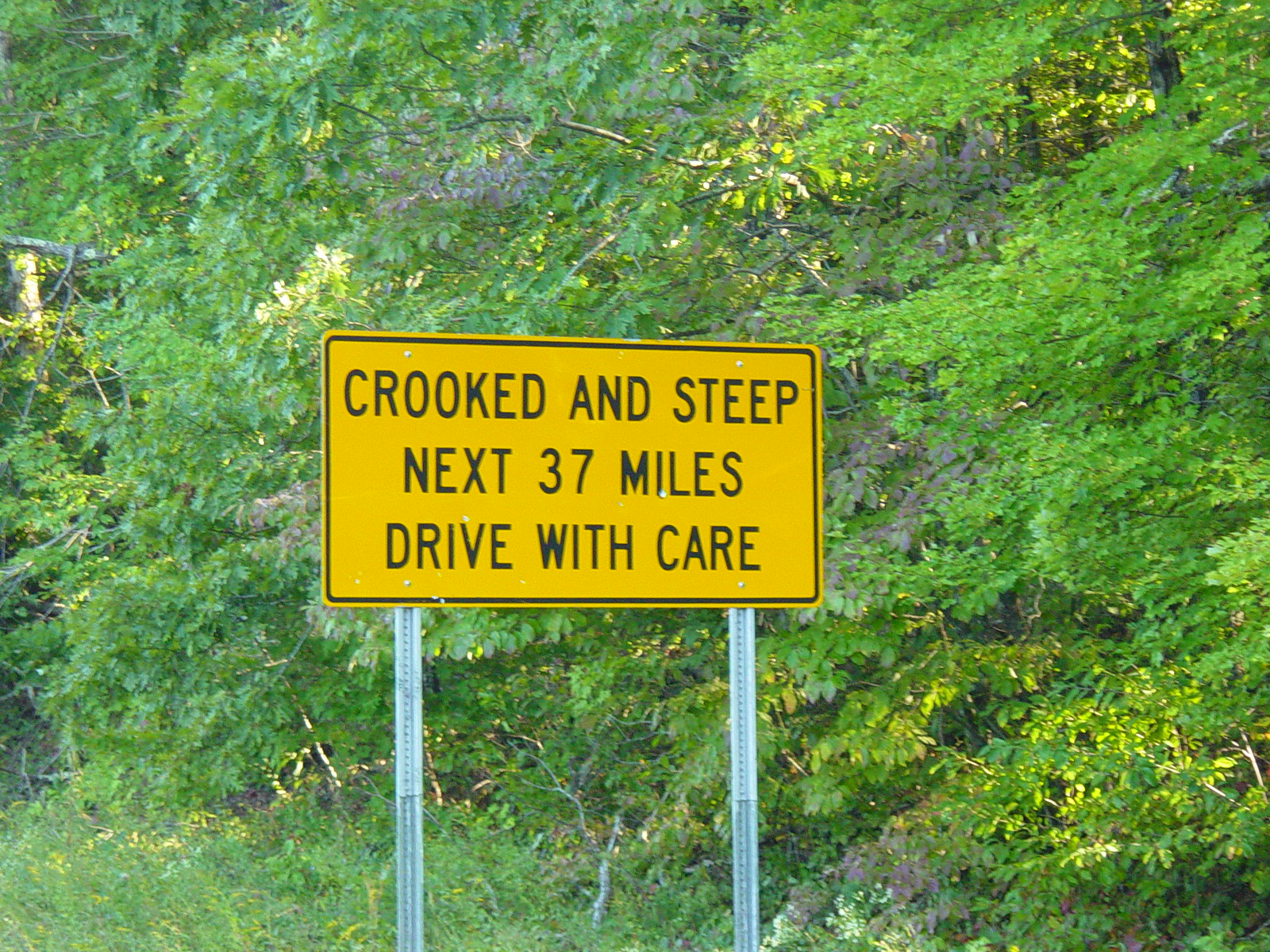The photograph features a rectangular, yellow road sign with a black border, prominently centered and occupying about a quarter of the image's height and width, excluding its supporting legs. The sign, mounted on two grey metal poles, bears a clear message in black, capital letters: "CROOKED AND STEEP," followed by "NEXT 37 MILES" and "DRIVE WITH CARE." Surrounding the sign is a rich, natural backdrop composed of numerous green trees and bushes, with some foliage displaying a mix of reddish and yellow hues. Sunlight filters through the branches, casting a gentle light across the scene, and long grass with sporadic yellow flowers grows at the base of the sign. The left side of the image also shows some greyish branches and a small, brighter area of sunlight peeking through.